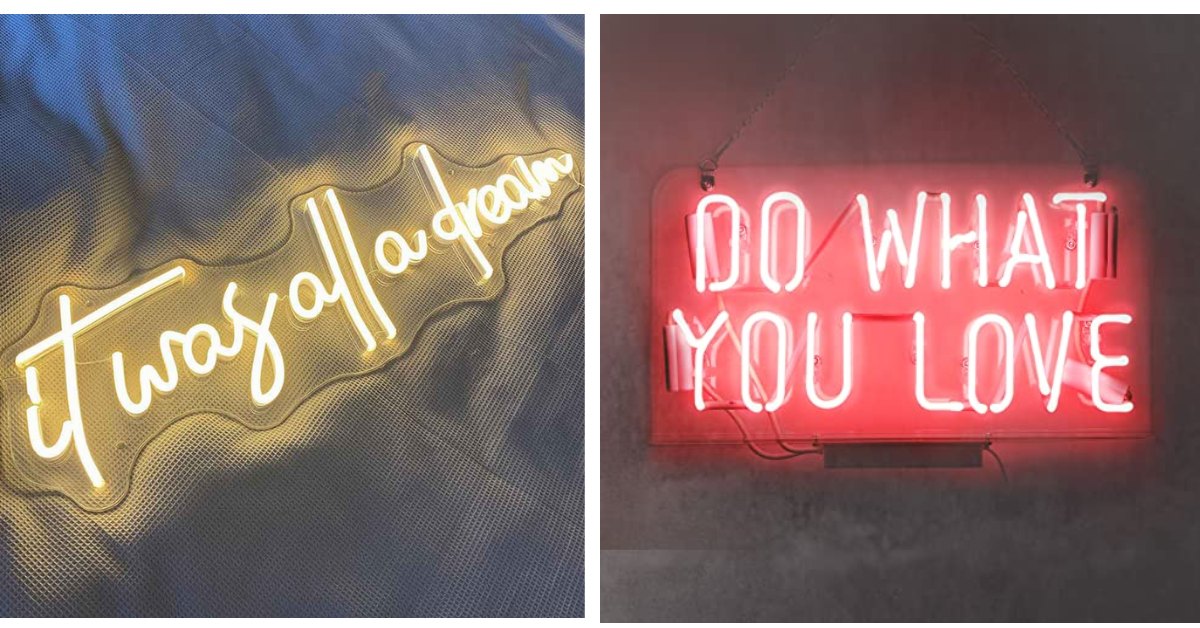The image features a side-by-side composition of two photos, each showcasing a neon light sign. On the left, a yellow neon sign diagonally rests on a wrinkled gray sheet or mattress, displaying the phrase "It Was All a Dream." On the right, centered against a purple background, a red neon sign with white, capitalized text reads "Do What You Love," arranged in two lines with "Do What" on the first line and "You Love" on the second. Both signs exhibit a cohesive artistic style, characterized by their vibrant colors – including yellow, red, white, black, gray, and hints of blue – and share a visually striking and artistic font, suggesting they were created by the same artist.